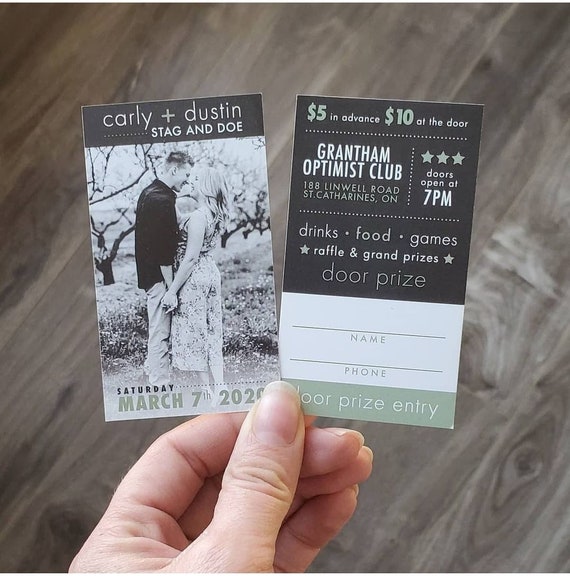The image displays a woman’s hand with unpainted long fingernails holding two small cards against a backdrop of a wood-grain floor. The cards, showcasing a monochrome black and white theme with a muted pistachio green accent, are the front and back design for an event invitation. The front card features a black and white photo of a couple, Carly and Dustin, about to kiss while holding hands with a scenic backdrop of trees, indicating a professional photo shoot. The text above the photo reads "Carly and Dustin Stag and Doe," with the event date, "Saturday, March 7, 2020," written at the bottom. The back card is primarily black with a white square for writing a name and phone number, designated for door prize entry. Additional details include the event location at the Grantham Optimist Club, 188 Linwell Road, St. Catharines, Ontario, with doors opening at 7 PM. Entry costs $5 in advance and $10 at the door. The card also lists event activities: drinks, food, games, prizes, raffle, grand prizes, and door prize.